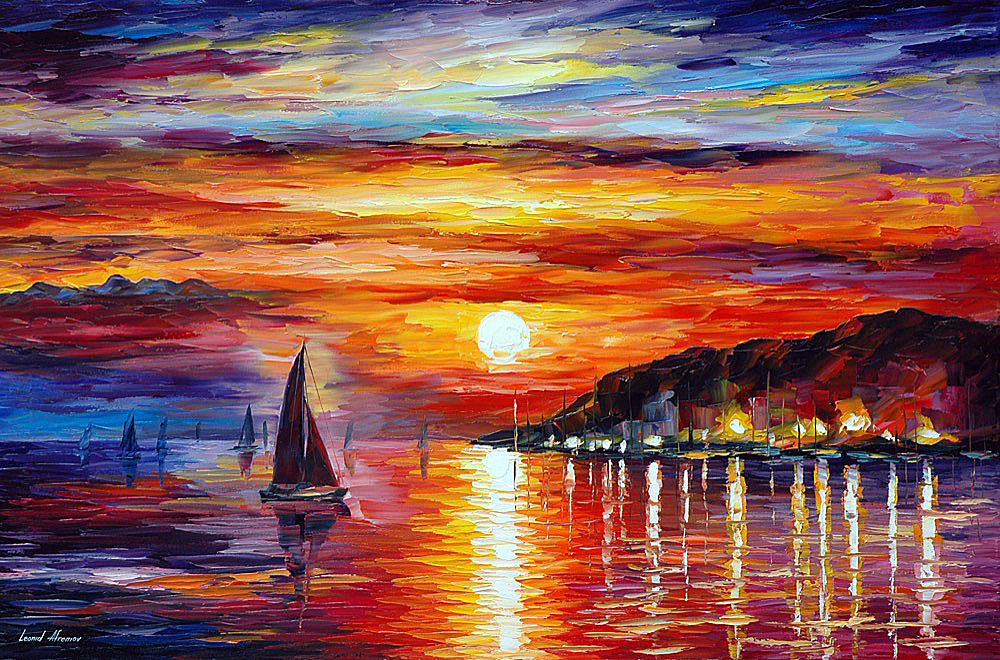The image is a vibrant and detailed painting of a boat harbor at sunset, likely created using a combination of oil paints and acrylic. Dominating the center of the painting is a bright, illuminating sun near the horizon, casting a radiant glow in a palette of yellows, oranges, and reds that transition into purples and blues towards the top of the sky and the edges of the painting. The water below captures a stunning vertical reflection of the sun, with the ripples shimmering in yellow and gradually blending into other warm hues.

The scene features several personal sailboats, around ten in total, scattered across the harbor, with their reflections beautifully mirrored in the water. Some of these boats are docked, their lights creating additional points of reflection on the surface of the bay. The thick, textured brush strokes and hints of palette knife work reveal a technique reminiscent of Van Gogh or Monet, enhancing the painting's dynamic and lively character.

On the right side, a rocky shoreline is depicted, adorned with small buildings that have lights illuminated, casting their reflections into the serene water below. In the bottom left-hand corner of the painting, the artist's signature can be seen in white, although it is too small to decipher. Overall, the painting intricately captures the peaceful yet vivid essence of a sunset over a bustling harbor.